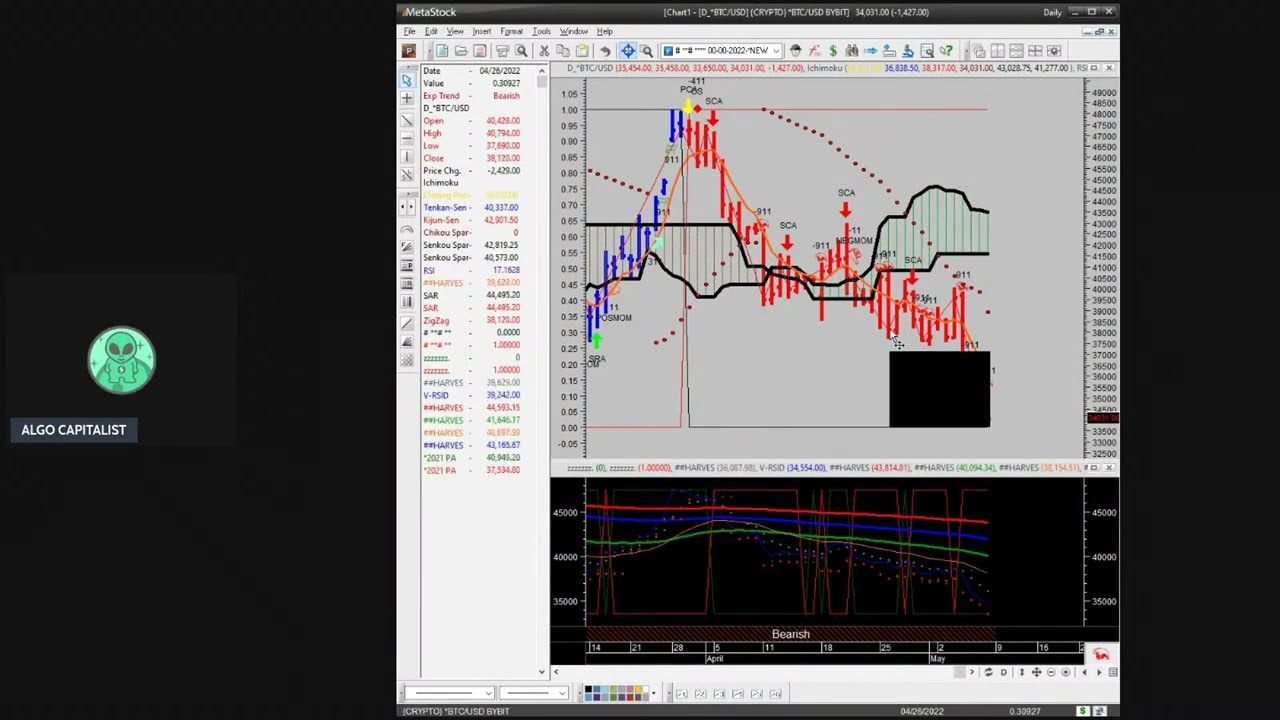The image is a detailed screenshot of a computer screen displaying a stock analysis program, showcasing various types of graphs and market indicators. Dominating the center is a large, detailed line and bar graph with blue, red, and yellow markings, illustrating trends and data fluctuations. This graph appears under the heading "MetaStock" and features multiple arrows pointing up and down, and annotations like "SCA" and "bearish," indicating market trends and patterns. Beneath the main graph is another line graph with red, blue, and green lines, highlighting additional data patterns.

The screen also includes a black background on the left, punctuated by a small, circular alien logo with the text "Algo Capitalist" in white, all caps beneath it. The left side of the screen is filled with numerous small numbers and different colored annotations, which are part of the stock analysis details. Despite their tiny size, they represent critical data points on both the x and y axes of the graphs. In summary, this image provides a comprehensive view of a complex stock analysis tool, complete with colorful graphs, trends, market sentiments, and a detailed numerical representation of stock market data.